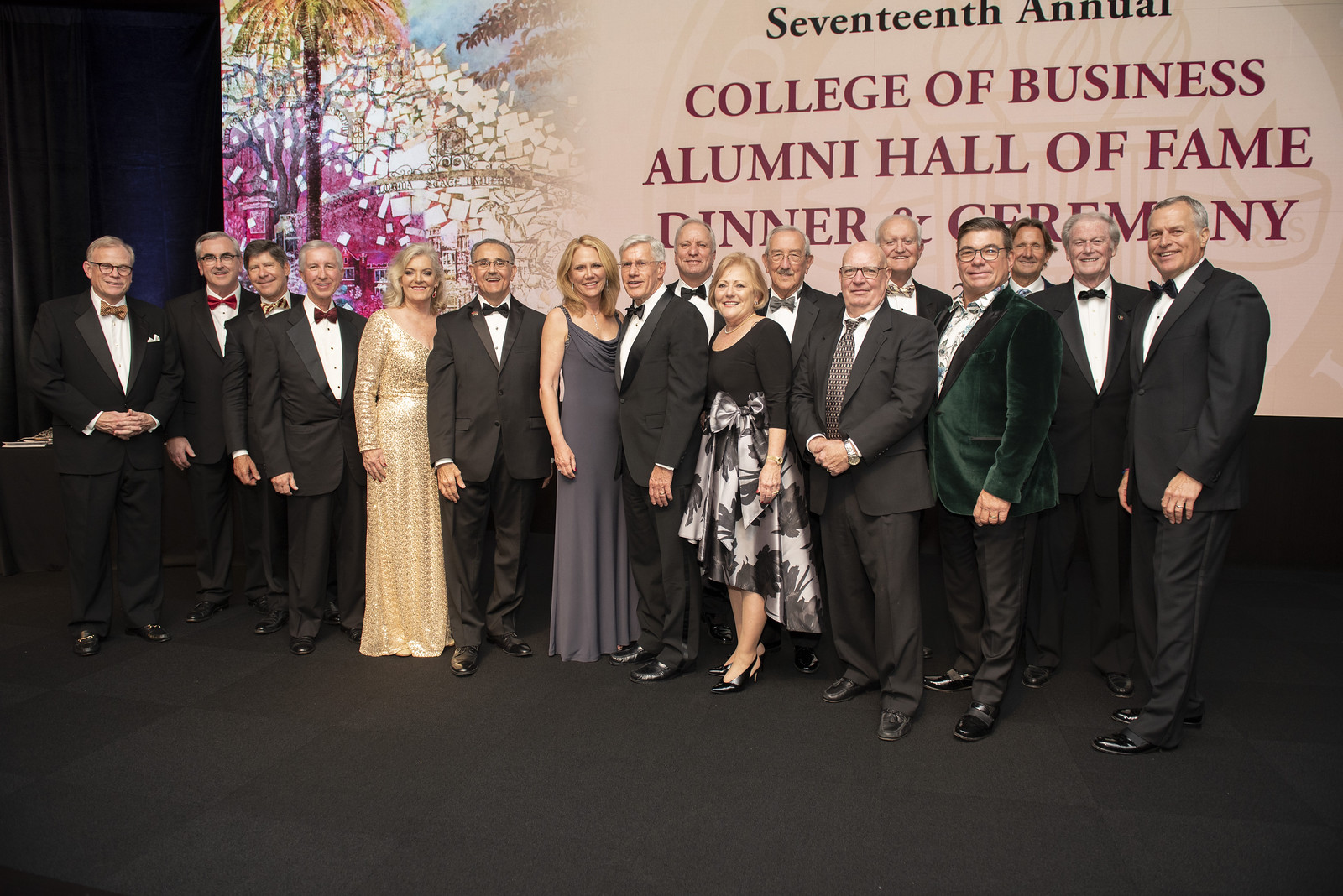The image showcases a group of 17 people arranged on a black stage, posing for a photograph at what appears to be the 17th Annual College of Business Alumni Hall of Fame Dinner and Ceremony. The majority of the individuals are men dressed in tuxedos or suits, with many sporting bow ties in various colors. There are three women in elegant dresses who are positioned more centrally within the group. The background features a large screen displaying the event details, though parts of the text are obscured by the individuals' heads. Notably, the stage is characterized by a black floor, and behind the group, there are some trees and palm leaves adding a touch of greenery. Most of the people are smiling, with a few adopting more neutral expressions, and while some have their hands clasped in front, others have their hands down by their sides.